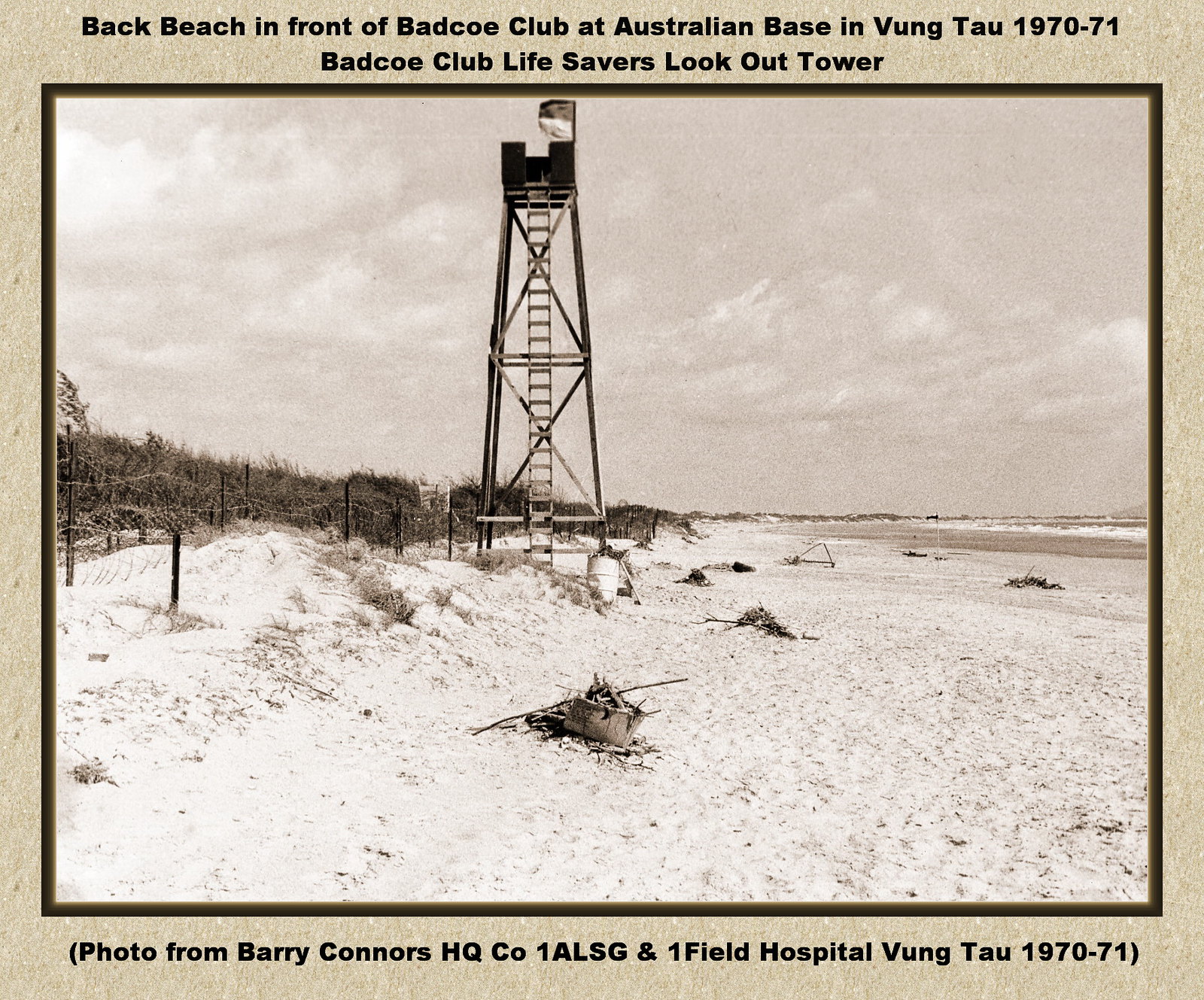This sepia-toned image, a historical photograph from 1970-71, showcases the Back Beach in front of the Badco Club at the Australian base in Vung Tau, Vietnam. Captured by Barry Connors, HQ CO 1ALSG in Onefield Hospital, the scene depicts the Badco Club Life Savers Lookout Tower prominently in the center. The rickety, flag-topped tower, accessible via a long wooden ladder, stands amidst a sandy beach. The ocean waves roll in from the right, while the left side is dotted with trees and shrubbery. The sky overhead is mostly cloudy, casting a subdued light over the scene. Strewn across the beach are remnants of boats and deliberate piles of brush. The image's brown border frames black text that provides context, detailing the location and significance of this lifeguard observation point.